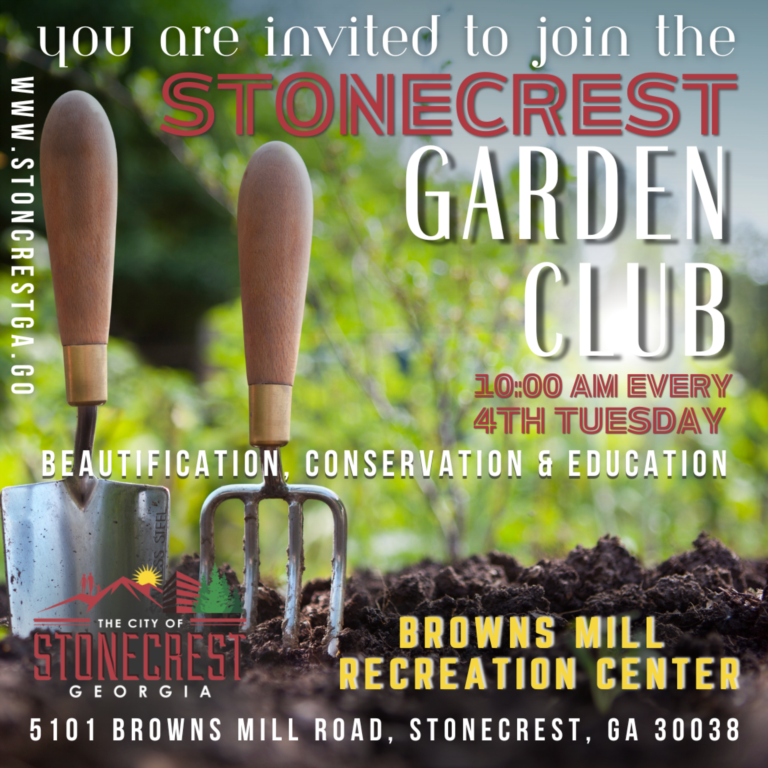The image is a square-shaped promotional picture, approximately six inches by six inches, inviting viewers to join the Stonecrest Garden Club. At the top, in eye-catching text, it reads, "You are invited to join the Stonecrest Garden Club, 10 a.m. every fourth Tuesday." Below this, the words "Beautification, Conservation, and Education" are prominently displayed. The bottom third of the image is dominated by tilled brown soil, into which a small hand shovel and a hand rake—both with wooden handles—are firmly planted. These tools suggest active gardening and community involvement. To the left, the website "www.stonecrestga.gov" is printed vertically. The background includes blurred green plants, adding a lush feel, and the upper right corner reveals a patch of blue sky. In the lower left-hand corner, there's an image depicting a cityscape with a tree and mountains, labeled "The City of Stonecrest, Georgia." Adjacent to this, in yellow, it says Browns Mill Recreation Center, and below it, the address "5101 Browns Mill Road, Stonecrest, Georgia, 30038" is clearly marked.